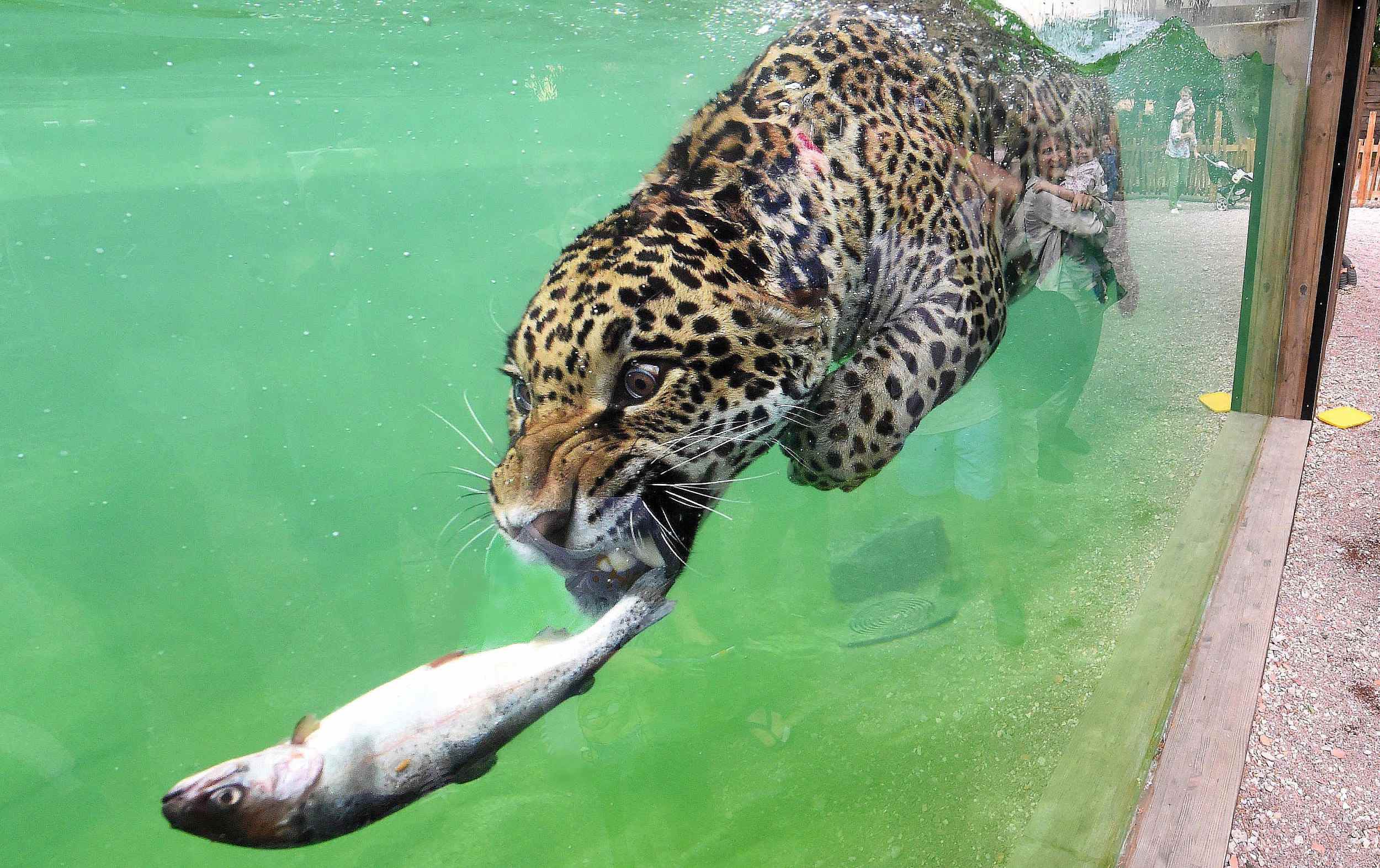The image captures a dynamic scene set in a zoo, featuring a close-up of a jaguar swimming underwater in a large aquarium tank with sea-green water. The jaguar, distinguished by its pale golden brown fur adorned with black spots and patches, is in the act of catching a fish, which is already in its mouth, showcasing its sharp teeth and whiskers. Reflected in the glass wall of the aquarium, a woman holding a smiling baby, presumed to be her grandchild, is visible. Additionally, there is a figure with a child on their shoulders and a stroller, seen further in the background.